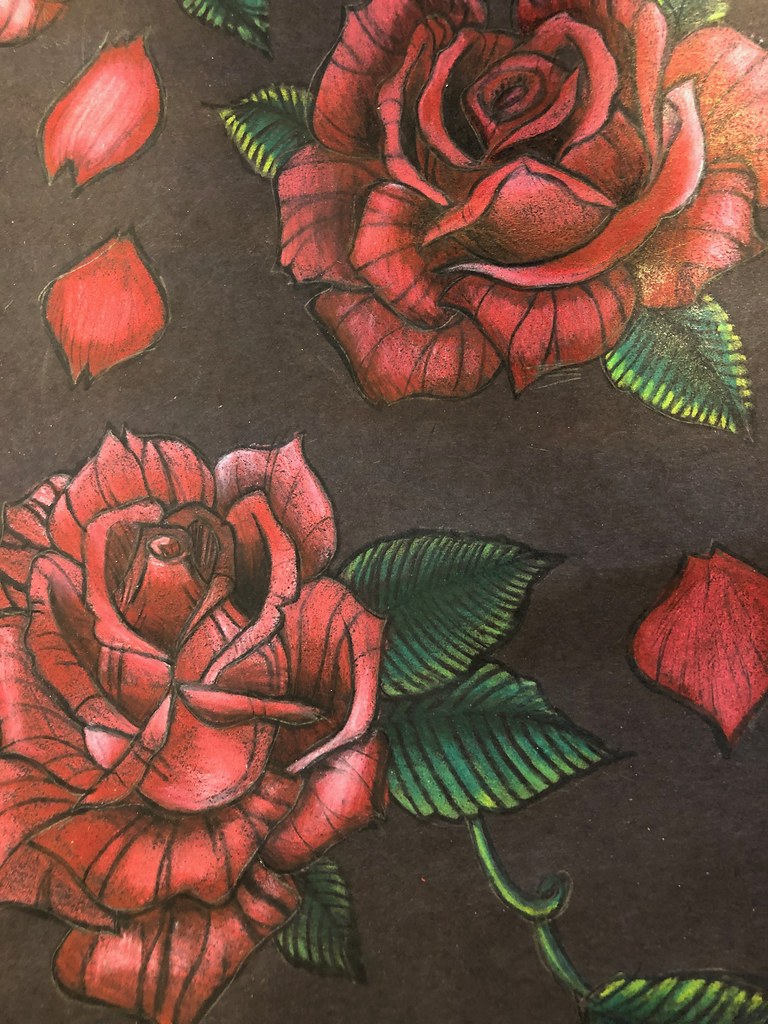This detailed pencil drawing of vivid red roses is set against a soft gray background. Featuring two fully open roses, one nestled in the top right corner and another in the bottom left, each bloom is about the size of a hand. The petals are richly shaded, with delicate white highlights imparting a realistic touch. Each rose is accompanied by green leaves, detailed with black veins and hints of yellow at the edges— the top rose has two leaves, while the bottom rose displays three. An artful stem curls dynamically between them, branching out with a curly Q and extending slightly off the page. Adding to the composition's depth, a few fallen rose petals are scattered on the ground, enhancing the sense of naturalism. The background is a dark gray canvas, contributing to the drawing’s striking contrast and overall aesthetic. No artist's signature is visible on the artwork.